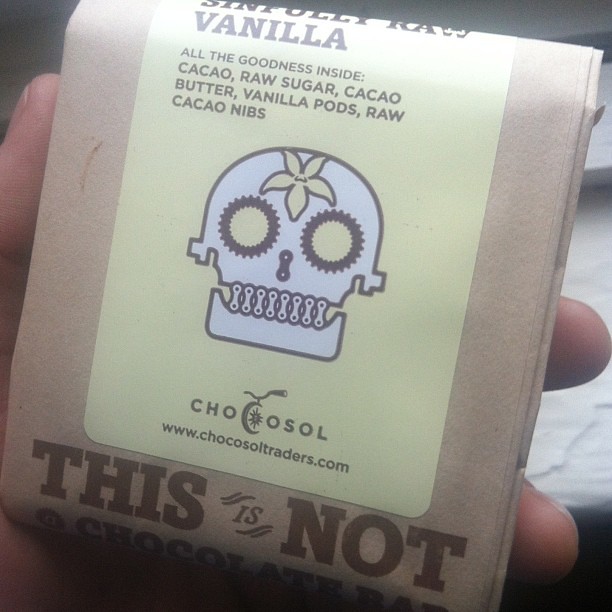The image features a close-up of a light brown package held in the hand of a Caucasian person, with only their fingers visible at the edges. The package is adorned with a large sticker that has a light greenish-yellow background with brown text. The label prominently displays the phrase "Sinfully Raw Vanilla" at the top, though the edge of the text is slightly cut off. Beneath this heading, there is an ingredient list that includes cacao, raw sugar, cacao butter, vanilla pods, and raw cacao nibs. Centrally positioned on the label is an artistic skull graphic, embellished with a flower on its forehead. Just below this skull, the brand name "ChocoSol" appears, followed by the website "ChocoSolTraders.com." At the very bottom of the label, partially cropped out, the text reads "This is not a chocolate bar." The background is dimly lit, with indistinct white objects that might be a table or similar surface.